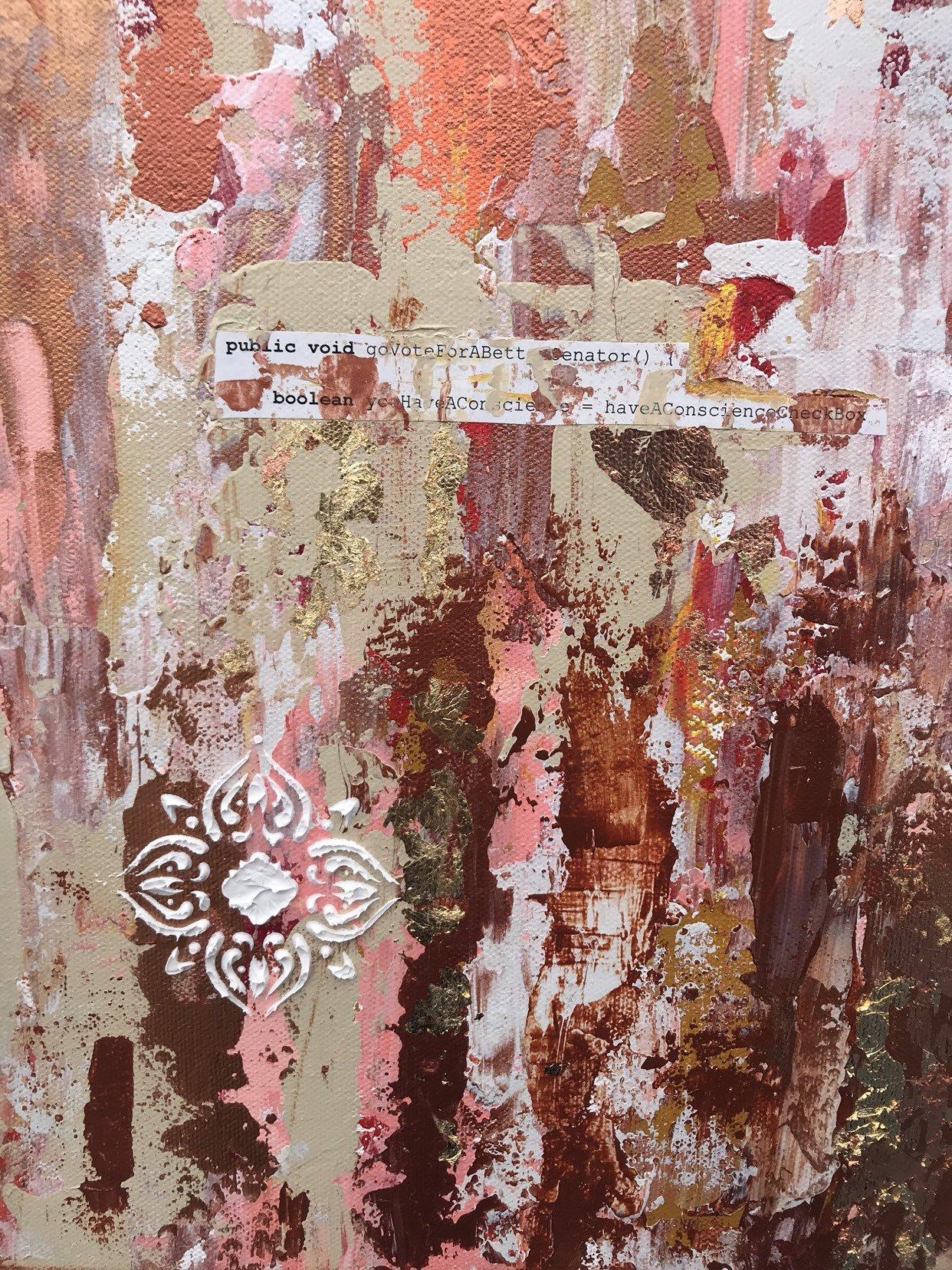This abstract painting features a textured mix of colors and mediums, predominantly showcasing a palette of neutral tones, soft peaches, pinks, and varying shades of bronze and brown. A tan-colored base layer of paint serves as the foundation for a composition of vibrant brush strokes, including coral, white, brown, reddish-brown, gold, and yellow hues, which blend and layer across the piece. Towards the upper center, a strip of white paper is glued onto the canvas, bearing the bold, lowercase text: "public void, go vote for a better senator." Below this, the partially obscured text reads "Boolean, have a conscience," with a checkbox indicated next to it. The bottom left corner features a white floral stamp, adding another layer of texture to this multi-faceted artwork. The piece is rich in visual depth and message, emphasizing call-to-action themes through its artistic expression.